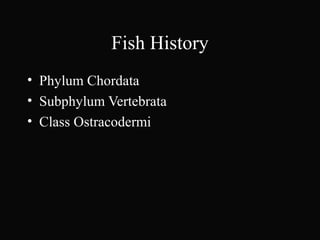The image features a small, black rectangle with the dimensions of approximately 1.25 times wider than its height. Centered near the top edge, the title "Fish History" is displayed in white capital letters, resembling a Times Roman font. Below the title, slightly off-centered to the left, are three bulleted points in white text. The first bullet point reads "Phylum Chordata," the second reads "Subphylum Vertebrata," and the third reads "Class Ostracodermy." The text and bullet points occupy the upper section of the rectangle, leaving the bottom half and the right side of the image completely black and void of any additional elements.